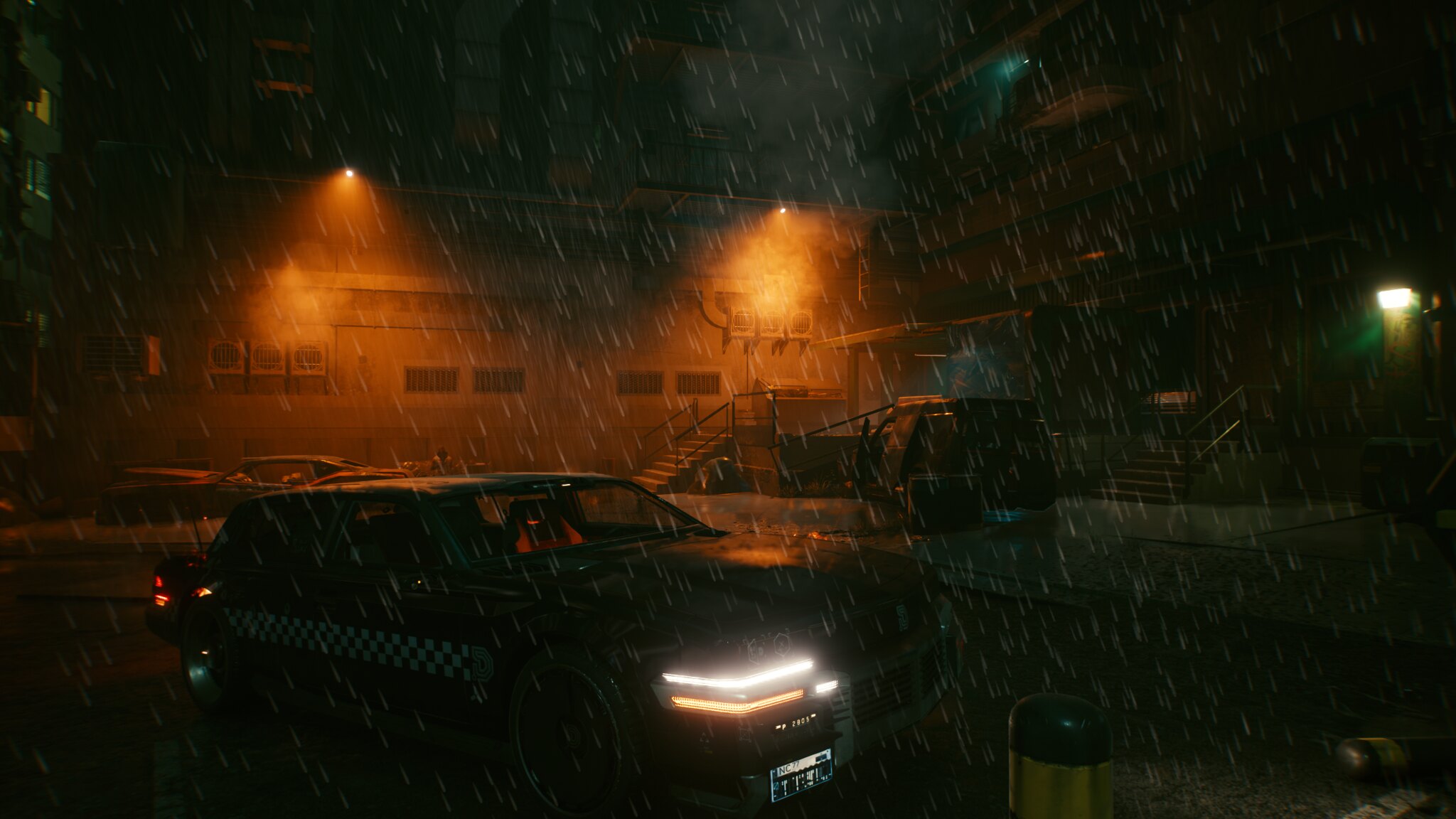A nighttime scene featuring a car positioned towards the lower right corner near a warehouse-style building. The building in the background is illuminated by several wall-mounted lights and features visible air ducts along its side. Adjacent to this building is another structure, forming an L-shape. In front of the building on the right, a van is parked with its rear facing the camera. The car closer to the camera, appearing to be a taxi, is distinguished by a black-and-white checkered pattern along its side. Its passenger-side headlight and taillight are both on, casting a glow in the dimly lit setting.